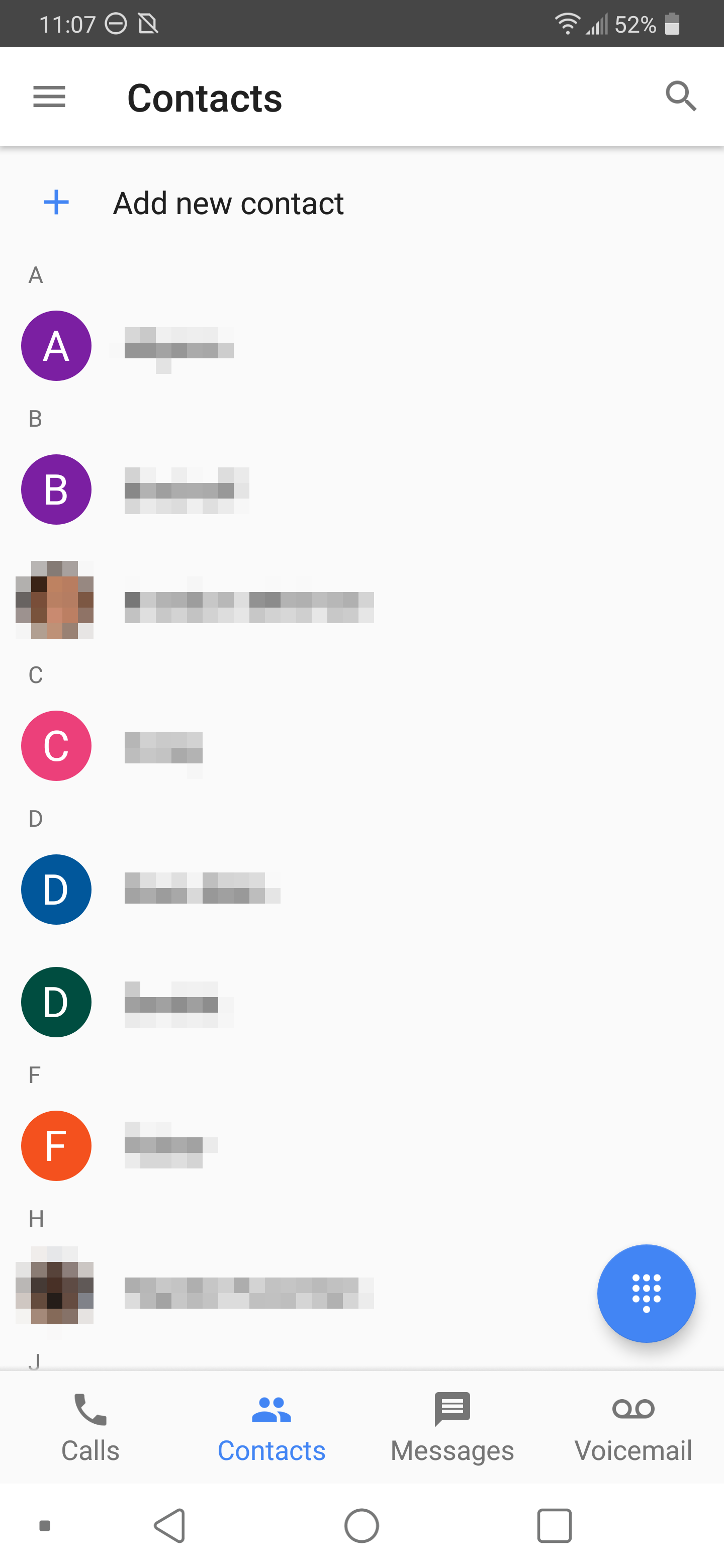The image is a screenshot from a cell phone, presented in a vertically elongated format approximately 2.5 times taller than it is wide. At the very top, the notification area is displayed as a horizontal black bar containing multiple elements. On the left side of this bar, written in white, is the time "11:07," followed by two unidentified icons. On the far right, there are icons for two wireless signals, a numeric indicator showing "52%," and a battery icon that appears to be approximately half full.

Immediately below the notification bar, the interface shows a menu structure. On the upper left, there's a hamburger menu (three horizontal lines), followed by the text "Contacts." On the far right of this section, there's a magnifying glass icon, indicating a search function. Below this menu section is a horizontal gray line separating it from the rest of the screen.

Further down, on the upper left, there is a blue plus symbol next to the text "Add new contact," which suggests that this is a contacts management page. The bulk of the image is taken up by a list of contacts, organized alphabetically by letter. Under the letter "A," there is one contact listed. The letter "B" has two contacts, "C" has one, "D" has two, "F" has one, and "H" has one. The contacts themselves are blurred, except for generic letter icons representing each contact.

At the bottom of the screen, a navigation bar contains standard buttons for "Calls," "Contacts" (which is highlighted in blue to indicate the current page), "Messages," and "Voicemail."